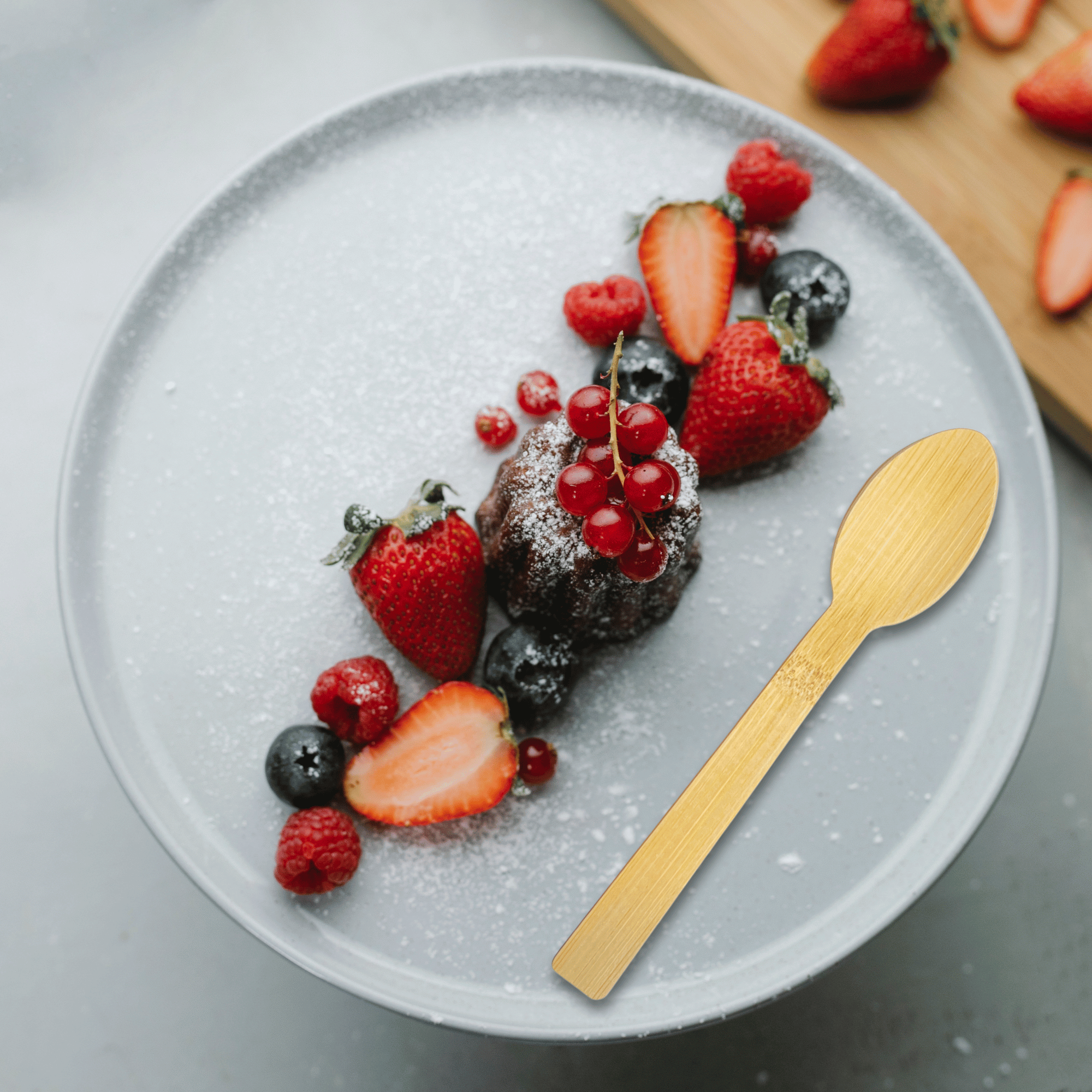The image features a close-up of a white plate set on a white table, adorned with an enticing arrangement of mixed berries, including blueberries, raspberries, strawberries, and possibly some dark grapes and red cherries. Some of the strawberries are halved, while a few remain whole with their tops still on. The fruits are artfully lined up in a straight line, and a light sprinkling of powdered sugar adds a touch of elegance to the scene. Adjacent to the berries on the plate is a light-colored wooden spoon, positioned parallel to the line of fruit. In the background, slightly out of focus, a cutting board holds additional strawberries, some of which are cut while others remain whole. This well-composed image captures the vibrant colors and textures of fresh berries, evoking a sense of freshness and delight.